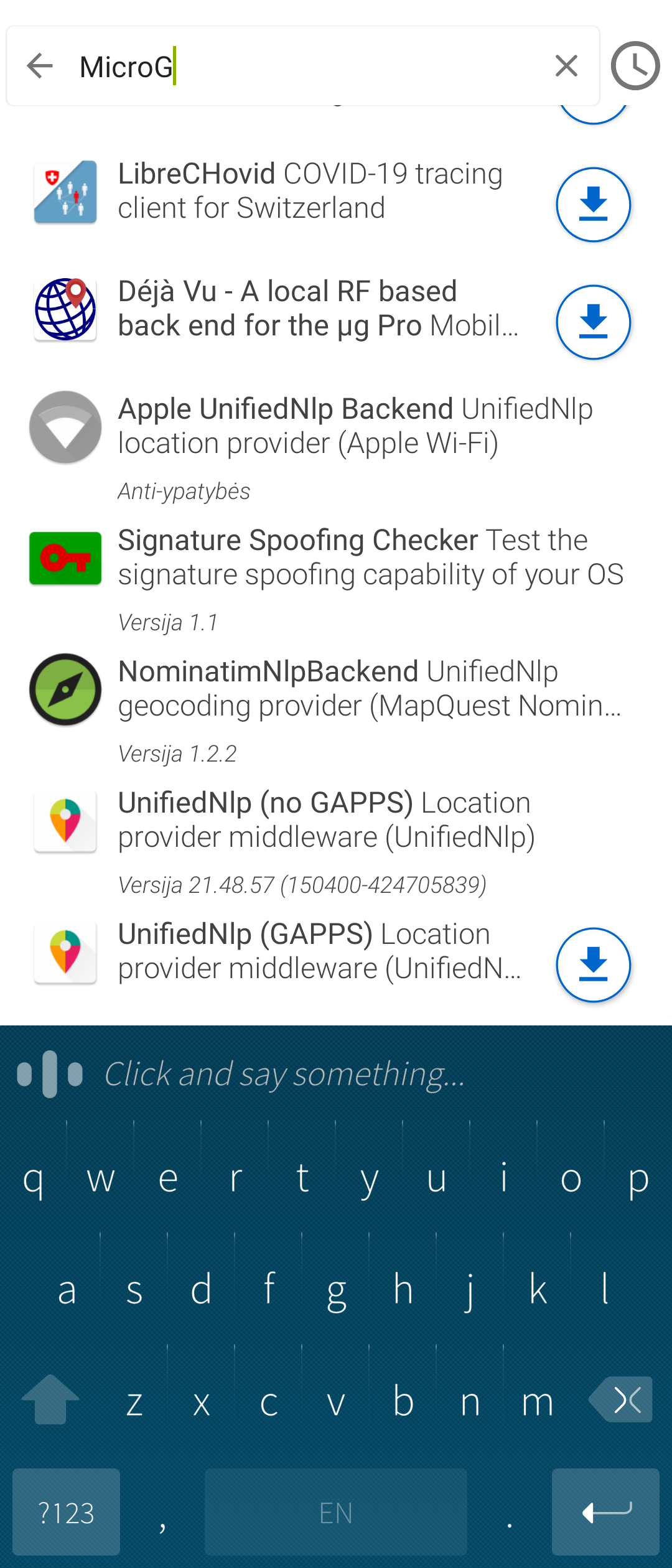In this image, we observe a screenshot of a mobile device displaying various apps related to location tracking and services. At the top, a search bar prominently reads "MicroG." Below the search bar, the first application listed is "Libre CHOVID," which is a COVID-19 tracing app specifically for Switzerland. Next, we have "Deja Vu," a local RF-based backend for MicroG's Unified Location Provider (UnifiedNLP). Following this is "Apple Unified NLP Backend," an app offering a Unified NLP (Network Location Provider) location service from Apple Wi-Fi data.

The list continues with the "Signature Spoofing Checker," designed to test the signature spoofing capabilities of the device's operating system, and "Mozilla NLP Backend," which is the Mozilla Network Location Provider. Then we see "Apple Wi-Fi," and "Name and Nature NLP Backend," providing another alternative location service.

Further down, there are entries for "Unified NLP Geocoding Provider" and "UnifiedNLP Location Provider Middleware," both integral components for location services on the device. Lastly, there is an entry for "UnifiedNLP GAPPS Location Provider Middleware," yet another location service provider. 

At the bottom of the screen, we see what appears to be a virtual keyboard typically found on a smartphone, suggesting that the user is actively engaged in searching or inputting data.